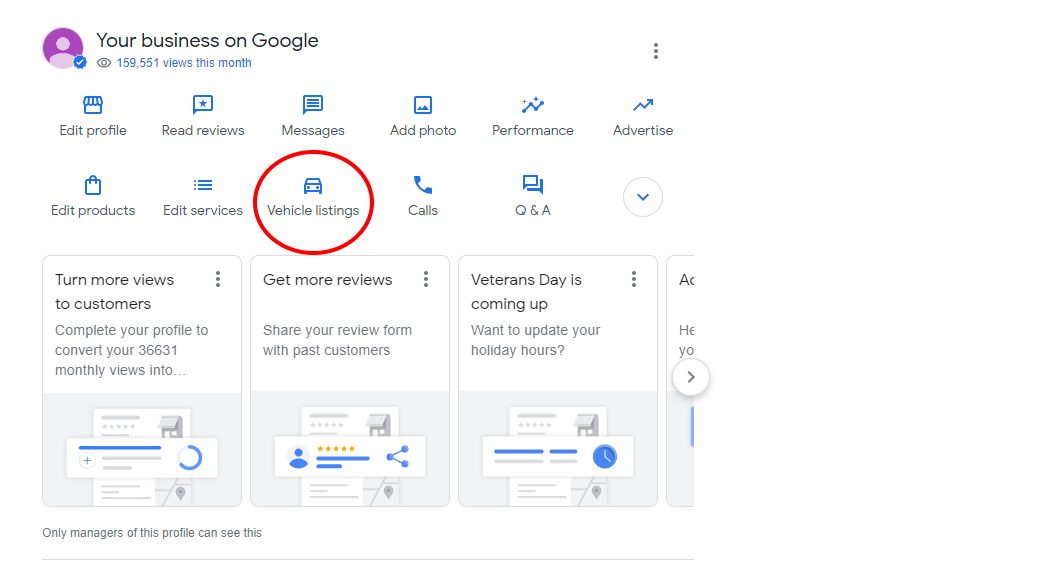In this detailed image of your Google Business screen, the top left corner features a purple profile icon. Adjacent to it, on the right, is the metric "Your business on Google, 159,551 views this month" displayed in small blue writing. Below this, there are two horizontal rows of categories, each represented by blue icons and black lettering. The top row includes: Edit Profile, Read Reviews, Messages, Add Photo, Performance, and Advertise. The bottom row features: Edit Products, Edit Services, Vehicle Listings, Calls, and Q&A.

The page is divided with a light gray background encompassing three main sections towards the bottom. In the white top half of the bottom section, the leftmost panel reads "Turn More Views to Customers," suggesting users complete their profile to convert the 36,631 monthly views into more meaningful interactions. The middle panel says "Get More Reviews" and encourages sharing the review form with past customers. The right panel reminds users that "Veterans Day is Coming Up" and prompts them to update their holiday hours. A fourth panel is partially visible on the far right, showing only about 10% of its content, suggesting that it is cut off from view. Everything in the image is set against a white background.

At the very bottom left, there's a note stating "Only Managers of the Profile Can See This," followed by a thin gray line stretching across the bottom from side to side, completing the image’s layout.